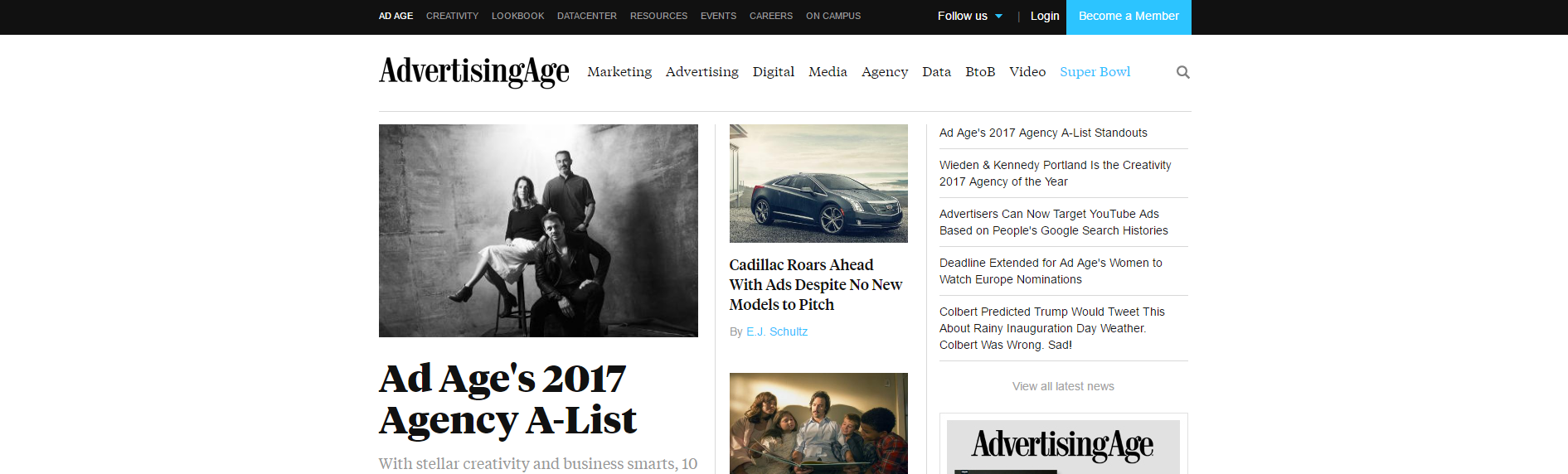This screenshot captures the interface of a magazine's website, showcasing a comprehensive navigation system. At the top of the page, the primary navigation bar features several clickable options designed to help users explore various areas of content. Key sections such as Digital Media, Agency, Data, and Video are prominently listed within the application menu situated on the left side, just below the bold, black bar that contains the website's title, "Advertising Age."

In the upper portion of the site, a light blue box highlights the members, drawing attention to registered users or featured personnel. At the heart of the image, there's a personal photograph depicting three individuals seated together, suggesting a moment of collaboration or camaraderie, adding a human touch to the digital interface. This detailed arrangement provides a clear and organized user experience, ideal for navigating the rich content offered by the magazine.